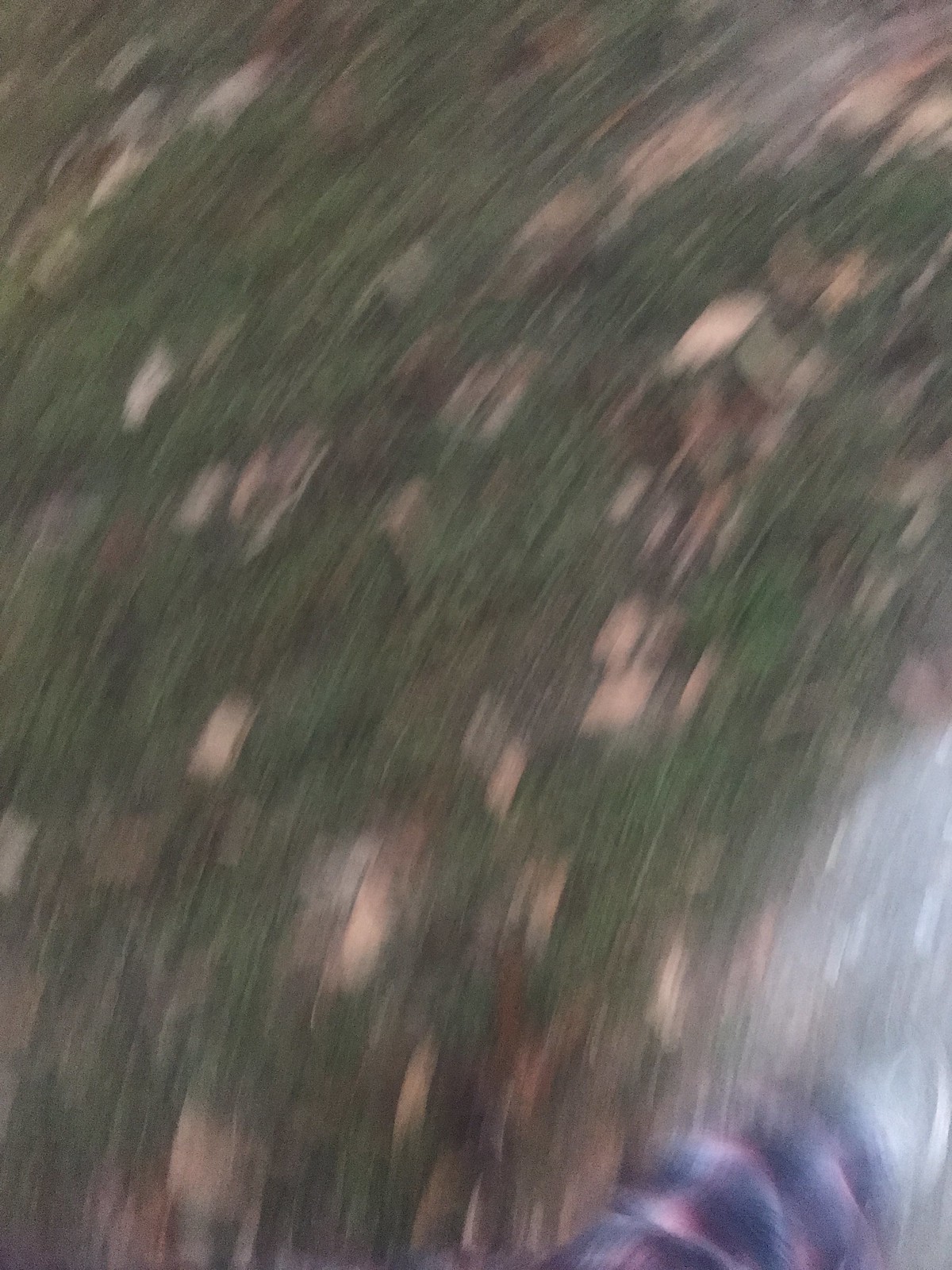This image is a vertically rectangular, excessively blurry photograph likely taken by accident. The motion blur creates a diagonal drag from the upper right to the lower left, giving the scene a dynamic but indistinct appearance. Predominantly, the image shows dark green grass scattered with numerous gray and brown leaves, suggesting a ground covered by autumnal foliage. In the bottom right corner, there is a partial, heavily blurred view of what appears to be the lower portion of a leg clad in pink, purple, blue, red, and white plaid pants, and a faint outline of a shoe, most likely a gray sneaker, standing on concrete or asphalt. Despite the image's significant blurriness, the details hint at the perspective of someone in motion, looking downward at the mélange of nature and the path beneath them.